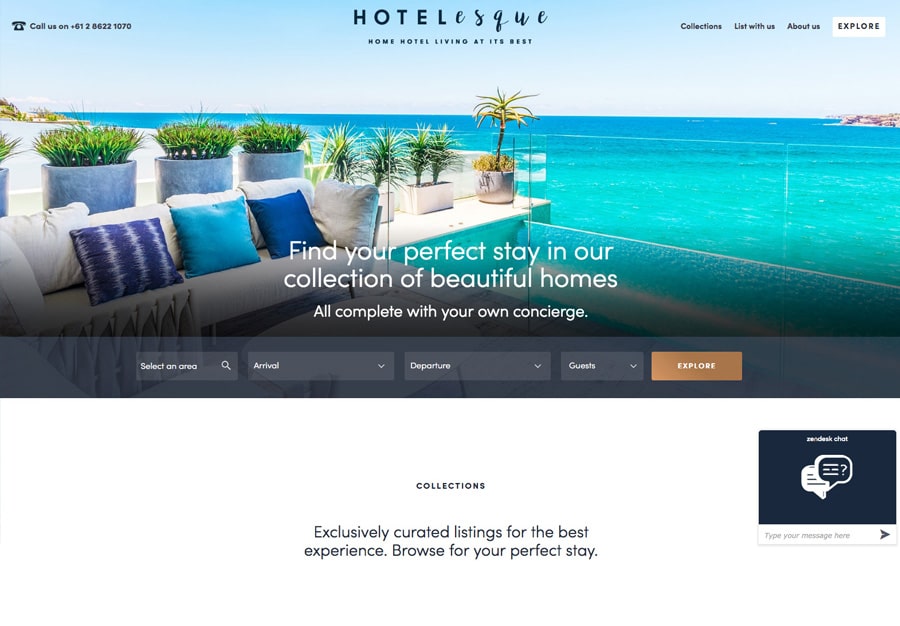Hotelesque - Discover Your Ideal Vacation Home

Explore our exclusive collection of beautiful homes with Hotelesque, where we offer a unique alternative to traditional hotels and resorts. On our homepage, you can find essential contact details on the left, such as our customer service number (612-8622-1070). Navigate through options on the right like Collections, List with Us, About Us, and Explore.

Centered prominently on the page, the Hotelesque logo is paired with our slogan: "Home Hotel Living at its Best." The backdrop features an inviting image of serene aqua-blue waters and a stylish beach setup—a cozy couch adorned with blue and purple pillows, surrounded by lush plants in large pots.

Search for your perfect getaway by selecting details such as area, arrival, departure, and the number of guests. For additional support, use our Zen Desk chat feature, marked by navy blue and white text bubbles with a question mark icon.

At the footer, explore our curated collections: "Exclusively Curated Listings for the Best Experience." Begin your journey to find the perfect stay with Hotelesque.